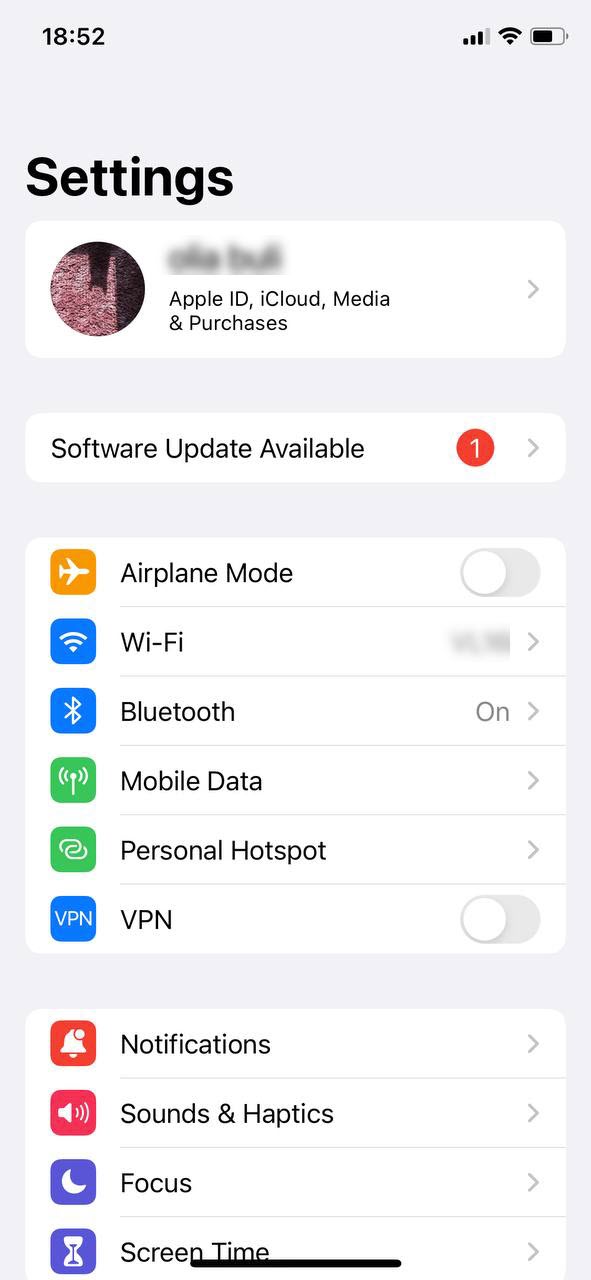The image shows a cell phone screen with the time displayed as 8:52. The top of the screen indicates cellular signal strength with bars and displays a three-quarters full battery icon. Below the time, there's a header labeled "Settings." Two words have been blurred out below this header, but the text "Apple ID, iCloud, Media & Purchases" is clearly visible.

A notification indicating a "Software Update Available" with a red circle displaying the number one is present; you can tap right to access it. Below, there are options for "Airplane Mode," "Wi-Fi," "Bluetooth," "Mobile Data," "Personal Hotspot," and "VPN." Among these, the Bluetooth feature is currently turned on.

Further down, settings for "Notifications," "Sounds & Haptics," "Focus," and "Screen Time" are visible. A black line divides the screen partway, separating the categories.

Icons are aligned to the left of each option: a plane for Airplane Mode, a Wi-Fi symbol for Wi-Fi, a Bluetooth symbol for Bluetooth, an antenna with lines for Mobile Data, two linked chains for Personal Hotspot, and the letters "VPN" for the VPN setting. Notifications are represented by a bell, Sounds by a speaker, Focus by a crescent moon, and Screen Time by an hourglass.

The image features a variety of colors including orange, blue, green, red, white, black, and gray.